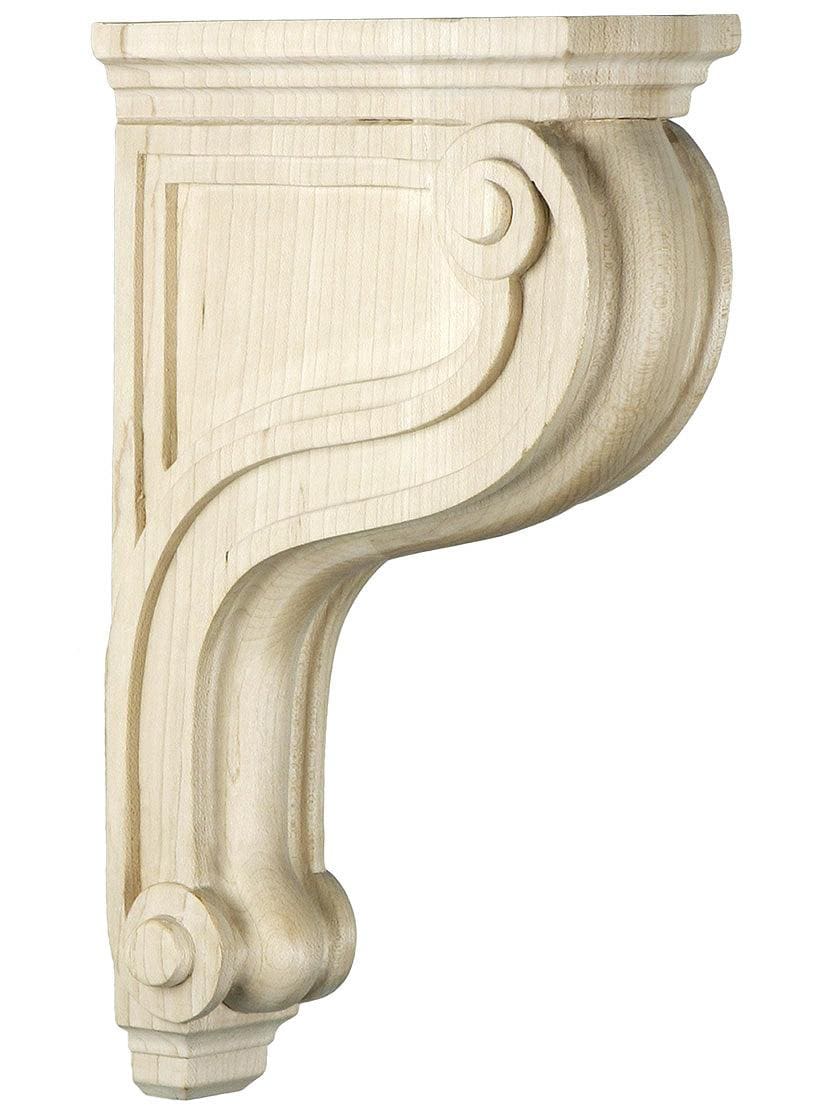The image depicts a decorative wooden corbel, intricately carved and unfinished or lightly finished in a light tan to white color, revealing distinct wood grain and vertical stripe patterns. Designed to enhance corners or support structures like shelves, the corbel features a flat top leading to a tiered section with three progressively shorter segments beneath it. The right side of the corbel curves outward before recurving back inward, creating a P-shaped silhouette. The central portion rounds downward into a smaller, tiered base. This piece, which could be mistaken for a bedpost leg, highlights detailed craftsmanship with square and line patterns along its edges, and decorative elements resembling bolts at both the top and bottom, making it an ornamental yet practical architectural accent.